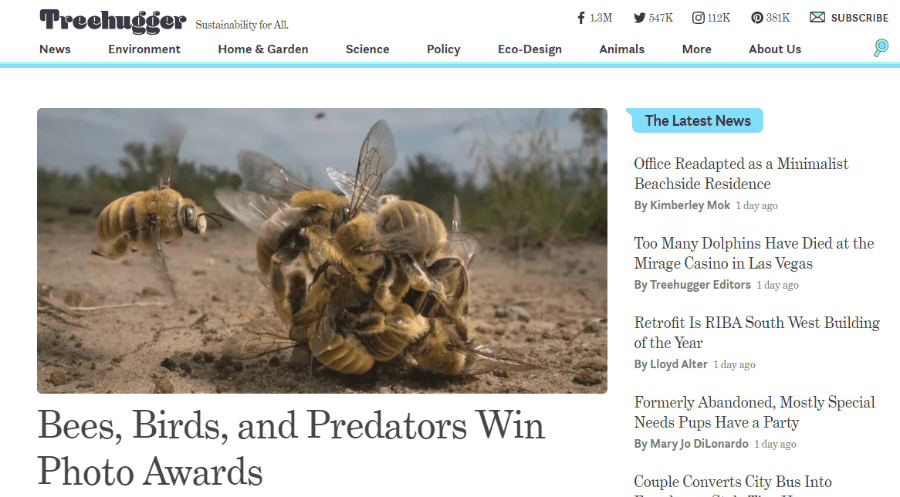The image is a screenshot from the Treehugger website, which has a white background. At the top, in bold print with a capital T, the site title reads "Treehugger: Sustainability for All." Below the title, social media icons for Facebook, Twitter, Instagram, and Pinterest are displayed, along with indicators showing the number of likes and followers. There is also a "Subscribe" option.

Directly underneath the Treehugger heading, a black navigation menu extends from left to right, featuring categories such as "News," "Environment," "Home & Garden," "Science," "Policy," "Eco-Design," "Animals," and a drop-down for "More" including "About Us." This menu is underlined by a turquoise line.

Beneath this, there is a photo displaying an outdoor scene with a background of sky, grass, trees, and dirt. A bee is flying in from the left side of the image, towards a clump of bees gathered in a ball. Capturing this moment, a caption reads "Bees, Birds, and Predators Win Photo Awards."

To the right of the photo, a turquoise banner with black text announces "The Latest News," followed by a list of different article headlines.